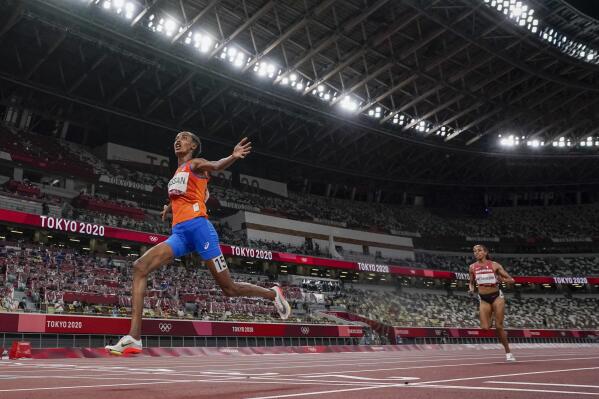This is a detailed photograph depicting an intense track and field race at the Tokyo 2020 Olympics, set in a packed, vibrant arena. The image captures two African-origin women, both athletes of exceptional speed and grace, racing against one another. The lead runner, identified by her orange tank top and blue athletic shorts, is airborne, seemingly having just leapt forward. She sports the number 15 on her leg and is wearing Nike athletic shoes. Her slender figure embodies both power and agility. Trailing a few steps behind her is another determined runner, distinguished by her red cut-off top that reveals her midsection and shorter black shorts, also wearing white athletic shoes. The background features a stadium brimming with spectators, rows of bright spotlights, and multiple displays of the "Tokyo 2020" logo, underlining the significance and global viewership of the event. The track itself is brown with marked white lanes, encapsulating the professionalism and excitement of this Olympic race.